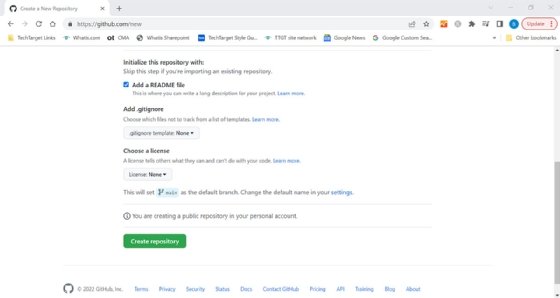The image depicts a blurry webpage with very small text, hosted on the GitHub website. At the top of the page is a light gray ribbon. On the left side of the screen, a tab labeled "Create a new registry" is open. The text beneath the gray ribbon is illegible due to its small size. The main portion of the screen, which has a clean white background, features a section titled "Initiate this repository with." Below this, there are options for "Add a README file" (which is checked), "Add .gitignore," and "Choose a license." At the bottom of this section, a prominent green button labeled "Create repository" is visible. Accompanying these elements is a gray scroll bar situated on the right side of the page.